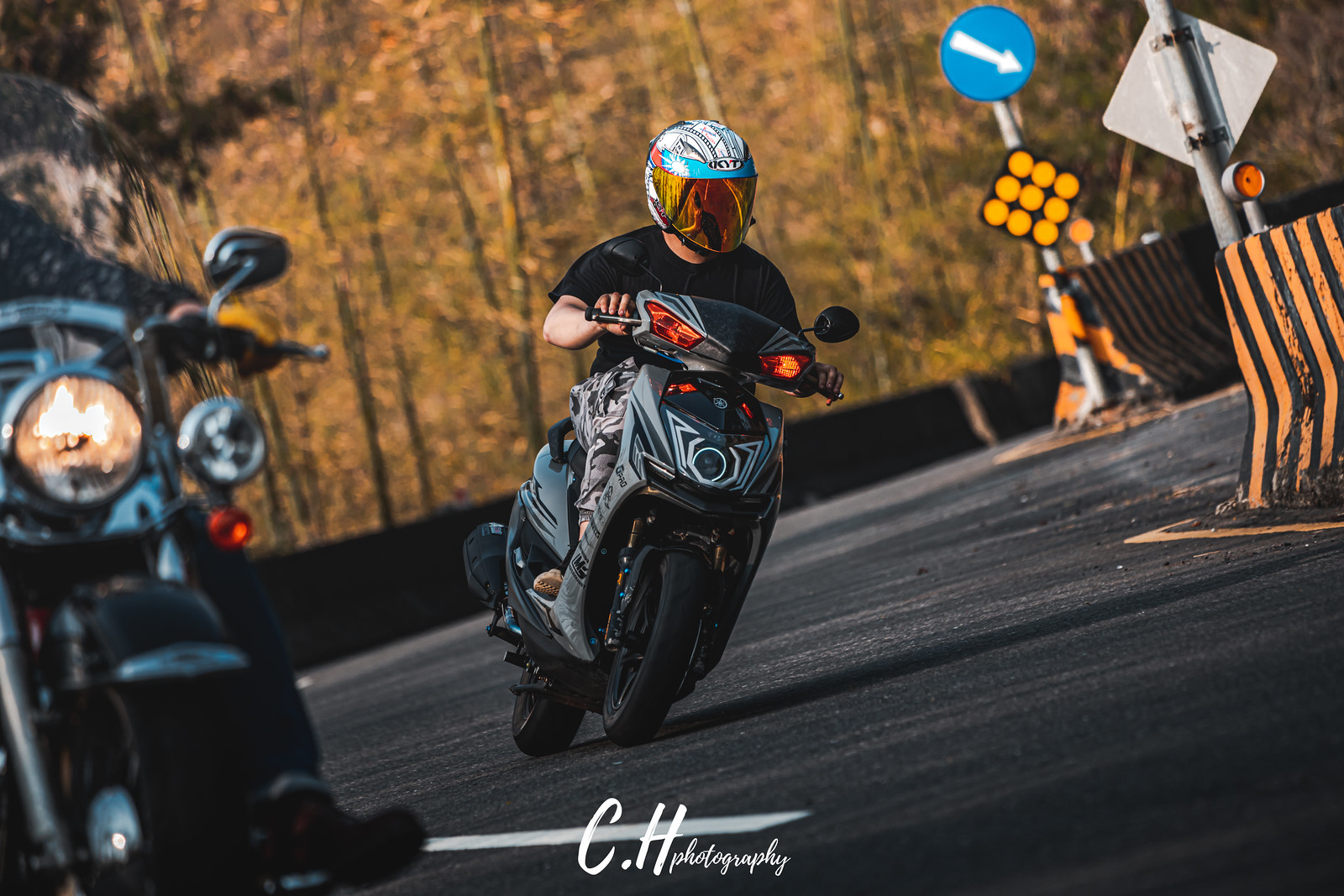A detailed photograph captures an outdoor scene on a seemingly new, paved racetrack flanked by yellow and black striped barricades and caution signs. The scene is set against a backdrop of a forest with tall, slender trees, glowing in shades of green and brown, suggesting a woodsy area. Dominating the right side of the image, a man dressed in a black t-shirt and blue jeans rides a black and gray motorcycle, his head protected by a striking white and blue helmet with graphical designs and a mirrored gold front face cover. He appears to be skillfully turning the motorcycle to the right around a corner. In the left foreground, another motorcycle with black and chrome details is partially visible, including the headlight, front tire fender, and the rider's dark shoe and blue jeans. Below center, a watermark in capital letters reads "C. H." with "photography" inscribed in small cursive font, indicating the professional credentials of the photographer.